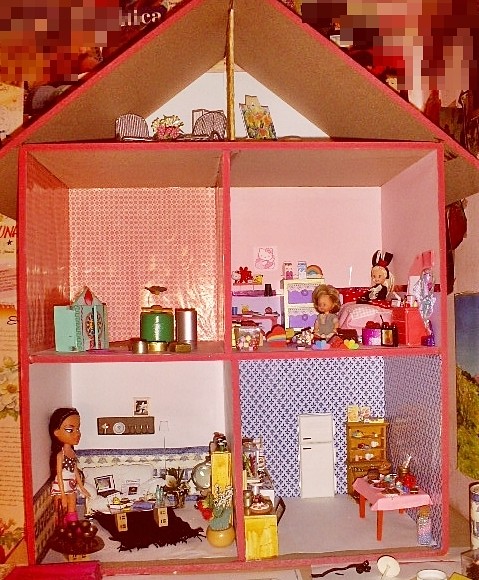This photograph depicts a large, vintage dollhouse with a brown sepia tone, likely from the 1970s, and constructed from thin wood. The dollhouse features an open design, revealing its intricate interior layout. It comprises four main rooms spread across two floors and an attic beneath a triangular roof. 

On the first floor, the bottom left room serves as a living room with a mother doll seated on a couch next to a black rug and various living room items. Adjacent to it on the right is the kitchen, equipped with a refrigerator, a table set with food, and a wooden shelf with drawers and dishes.

The second floor houses two rooms: the top right room is a bedroom containing two baby girl dolls on a bed, along with toys and dressers. The room on the left of the bedroom holds some indistinct objects.

The attic, located under the roof, contains chairs, flowers, and paintings, adding a touch of charm to the overall vintage aesthetic of the dollhouse. The colors within the house vary, with hues of pink, yellow, blue, red, white, and brown enhancing the miniature furnishings such as lamps, chairs, a dresser, and other household items.